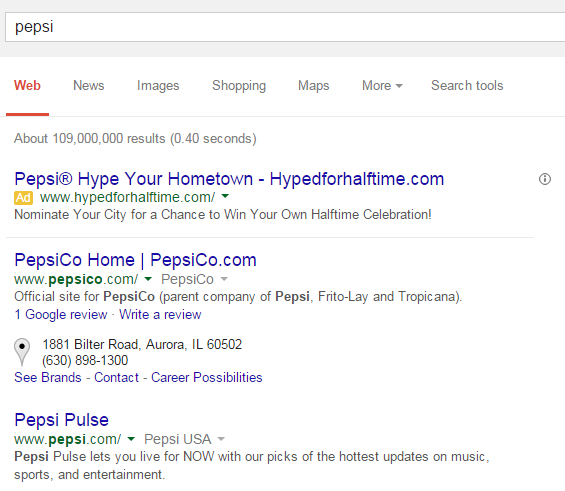**Detailed Description of the Search Engine Results Page for "Pepsi"**

At the top of the image, there's a white rectangular search bar outlined in gray, partially cut off on the right-hand side. Within this bar, the word "Pepsi" is typed in black font. Below the search bar is a gray section that indicates various search categories.

From left to right, the tabs read:
1. "Web" (highlighted in red).
2. "News" (black).
3. "Images" (black).
4. "Shopping" (black).
5. "Maps" (black).
6. "More" (black).
7. "Search tools" (black).

Below these tabs, there's a line of text in black displaying the number of search results: "About 100,000,000 results (0.40 seconds)."

The first search result is as follows:
- The title "Pepsi: Hype your hometown, HypeforHalftime.com" appears in blue.
- Below the title is a yellow box with the word "Ad" in it, and next to it in green is the URL "www.hypeforhalftime.com", followed by a downward-pointing green arrow.
- Below the URL, in black text, it says: "Nominate your city for a chance to win your own halftime celebration!"
- A thin green line extends across the bottom of this result.

The second search result is formatted as:
- The title "PepsiCo Home" in blue text.
- Beneath the title is the URL in green: "www.pepsico.com" along with a triangle pointing downwards.
- "PepsiCo" in gray color with the same downward-pointing triangle follows.
- Underneath, in black text: "Official site for PepsiCo, parent company of Pepsi, Frito-Lay, and Tropicana."
- Next is a blue text link: "One Google Review – Friday Review."
- Finally, in black text, the address "1881 Blitter Road, Aurora, Illinois, 60502."